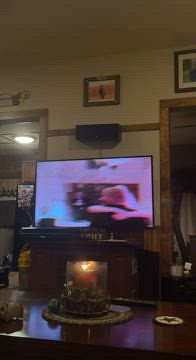A cozy living room scene is captured from a seated perspective on a couch. Central to the image is a coffee table adorned with a lit candle in an elegant candle holder, casting a warm, inviting glow. Against the pristine white wall stands a large flat screen TV, though the content on the screen is too blurry to discern. Above the television, a sleek soundbar is mounted, enhancing the audio experience. To the right of the TV, an open closet reveals neatly arranged clothes, adding a touch of lived-in comfort. On the left, an entryway or large mirror reflects light from an adjoining room, the source of which is a bright lamp. Completing the homely ambiance, several photographs in dark wooden frames are meticulously arranged above the TV, adding a personal touch to the decor.